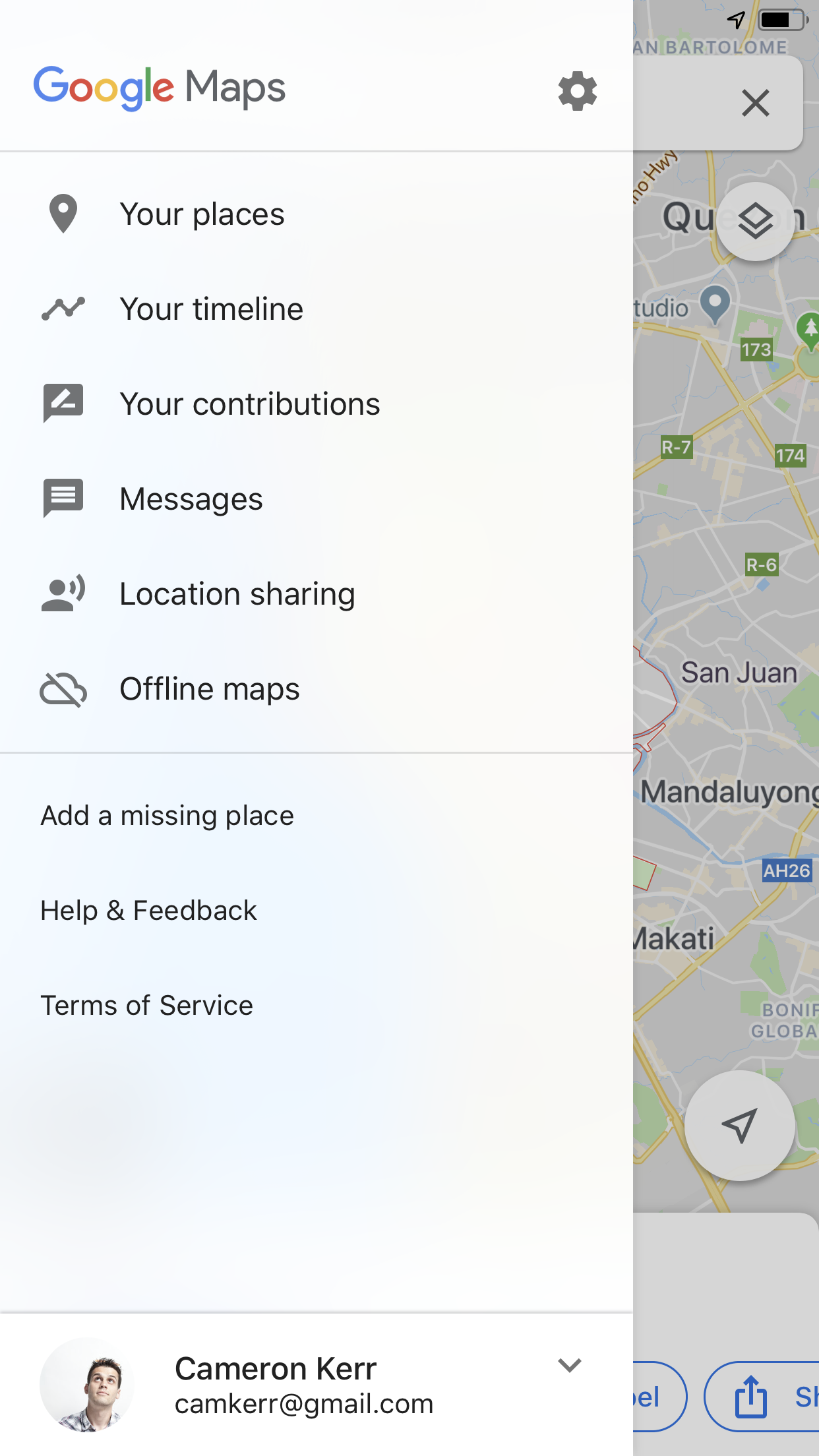This image is a screenshot from the mobile version of Google Maps. The background displays a map of a metropolitan area, featuring locations such as San Juan, Mandaluyong, and Makati. The map itself shows a grayish base color, highlighted with green areas representing parks or other green spaces, and yellow lines depicting roads. Labels identifying different places are marked in black text.

Dominating the screen from the left side and extending to most of the right side is a pop-out sidebar with a white background. At the top left of this sidebar, "Google Maps" is prominently displayed, while the top right features a settings icon. Below these, a list of options is presented in the following order: Your places, Your timeline, Your contributions, Messages, Location sharing, Offline maps, Add a missing place, Help & feedback, and Terms of service. At the very bottom of this sidebar, the user's information is visible, showing the name "Cameron Kerr" and the email address "camker@gmail.com."